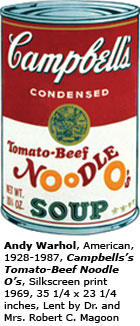This image prominently features an Andy Warhol art piece of a Campbell's Tomato Beef Noodle O's soup can. The artwork is a detailed silkscreen print from 1969, measuring 35 1/4 by 23 1/4 inches, lent by Dr. and Mrs. Robert C. Magoon. This print captures a quintessential 1960s-70s style and is rendered in Warhol's iconic hand-drawn aesthetic. The can showcases the top half with a distinct red background and the bottom half in white. The red section at the top displays the recognizable "Campbell's" in cursive script, followed by "condensed" underneath. Positioned where the red transitions to white is a small gold and blue medallion, emblematic of the Campbell’s brand. On the white part of the label, the text "Tomato Beef Noodle O's Soup" appears in a multi-colored palette of red, yellow, and green, with the O's resembling pasta in red sauce. Additionally, the can's net weight is specified as 15 1/2 ounces, and the image includes four silver stars. This piece by Warhol not only showcases the soup can but also highlights his ability to transform a commercial product into a celebrated piece of fine art.